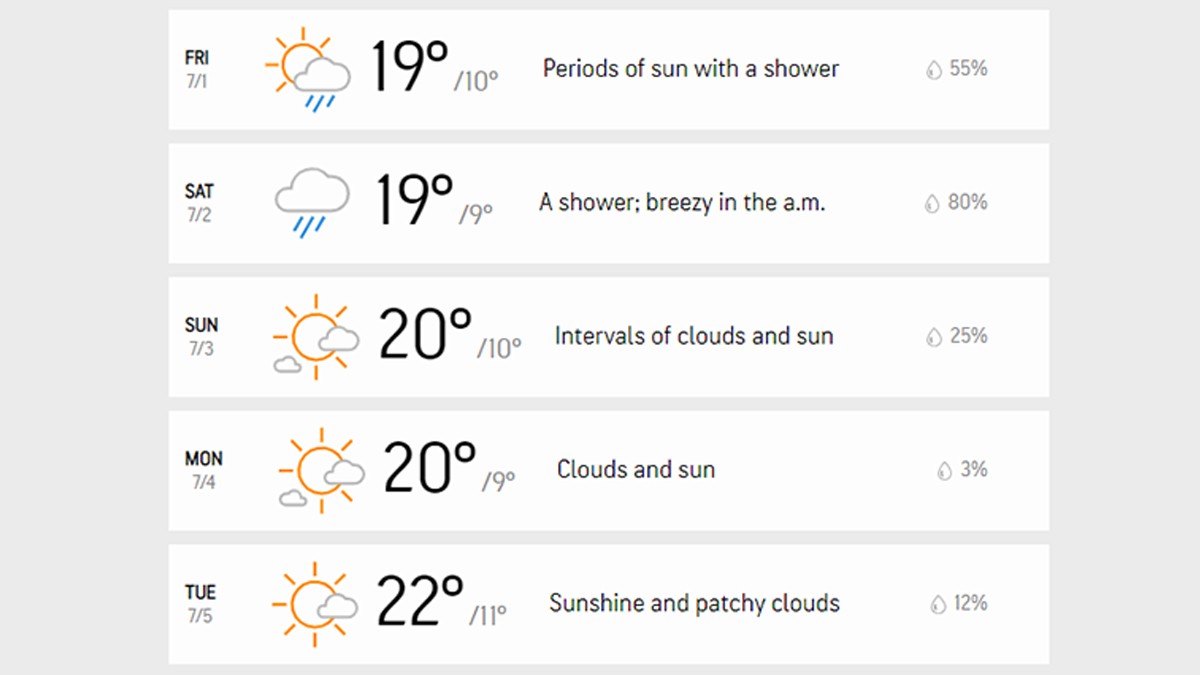This screenshot showcases a generic weather forecast covering the period from Friday, July 1st, to Tuesday, July 4th. Unfortunately, the specific location is not identified in the forecast. The dates are listed on the left side of the image, and the corresponding weather predictions are detailed alongside them. 

For Friday, July 1st, the forecast anticipates periods of sun interspersed with showers, with a high of 19°C and a low of 10°C. The chance of precipitation is noted at 55%, clearly marked in black text on the right.

Moving to Saturday, July 2nd, the weather is expected to be rainy and breezy in the morning. The high will be 19°C, while the low will drop to 9°C. The probability of precipitation is considerably higher at 80%.

On Sunday, July 3rd, the forecast predicts intervals of clouds and sunshine, with a high of 20°C and a low of 10°C. The likelihood of precipitation is lower, at 25%.

Finally, for Monday, July 4th, the weather will be similar to the previous day but with slightly different temperatures. The high will remain at 20°C, and the low will be 9°C. The chance of precipitation is marginally higher, at 30%.